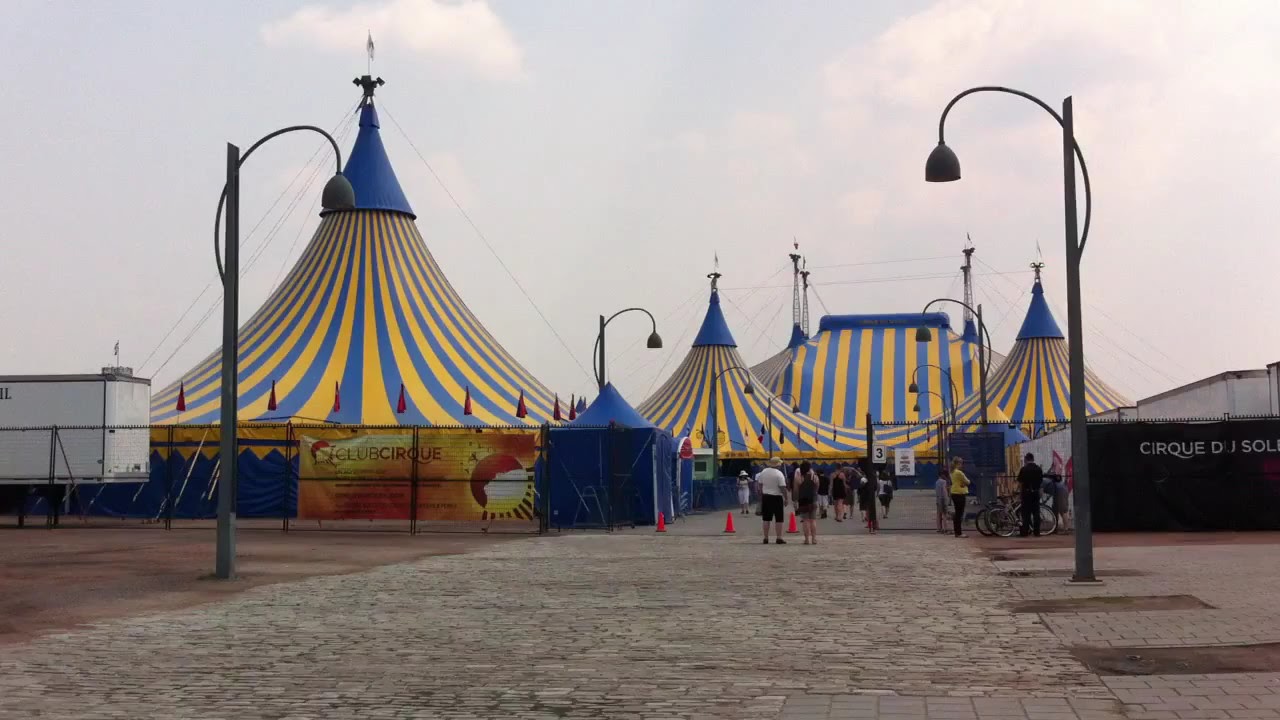The image depicts the lively entrance of a fairground, likely the Cirque du Soleil, taken during the daytime. The foreground of the picture showcases a stone and brick courtyard leading to the entrance, flanked by tall, vertical street signs with arched lamp posts on either side. The midline of the image features a tall chain-link fence adorned with posters; one on the left, vibrant in hues of yellow and orange, reads "Club Cirque," while the black poster on the right says "Cirque du Soleil." A group of people can be seen gathered near the open gate, marking the entryway.

In the background, there are four large tents. Three of these tents have peaked rooftops, adorned with spires and statues at the very top, while the fourth tent has a flat top. All tents are designed with vertical green, blue, and gold stripes cascading from their blue tops. To the right-hand side, there are some bikes with people gathered around them; to the left, pedestrians fill the walkway. The sky above is a light bluish-gray, dotted with a few clouds, adding to the overall ambiance of the scene.